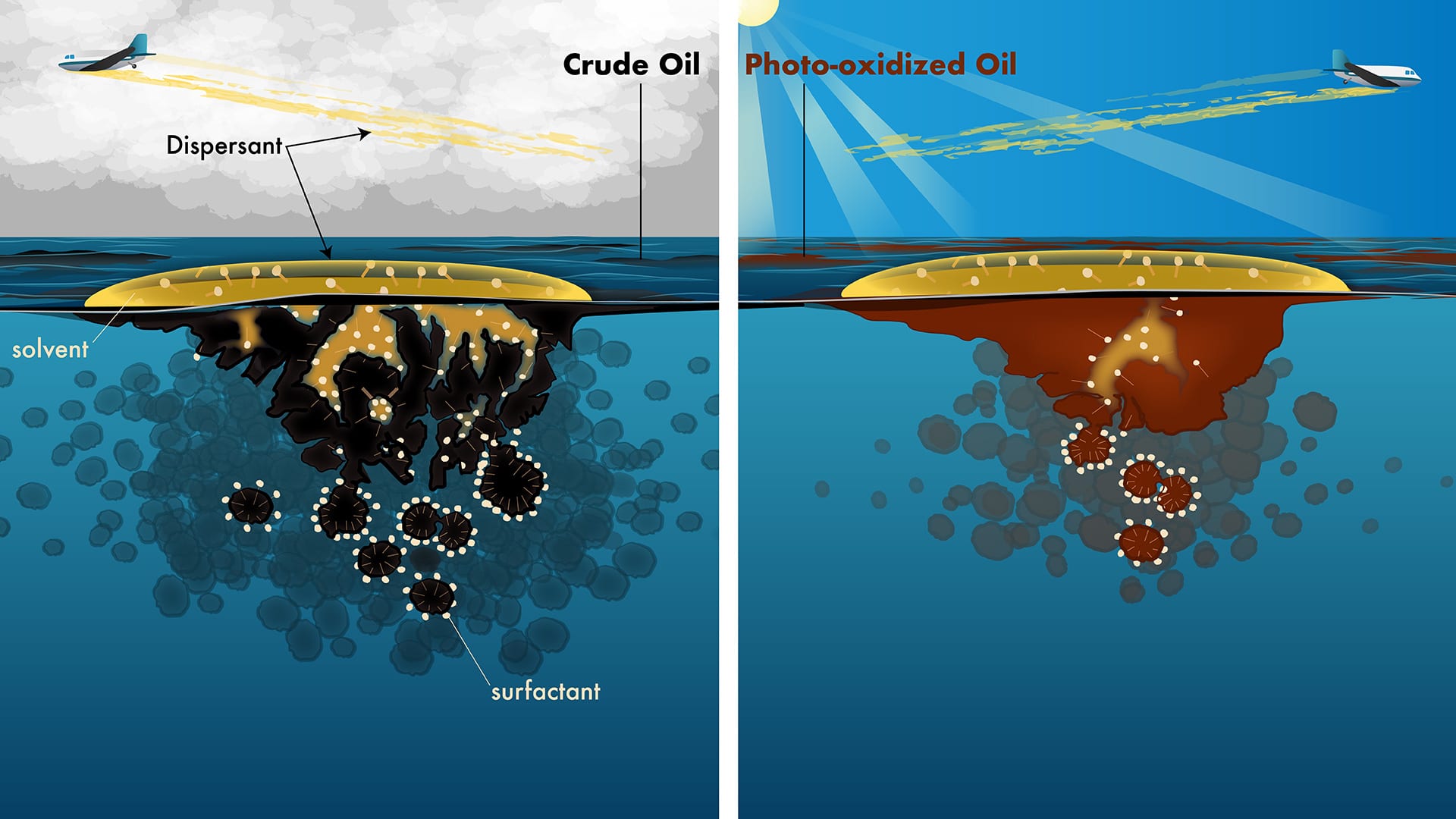The image consists of two detailed diagrams illustrating the process of cleaning up oil spills in the ocean. Both diagrams feature an airplane dispersing chemicals over the water's surface, symbolized by white aircraft releasing yellow streaks.

On the left, the diagram is labeled "Crude Oil and Dispersant" and depicts a cloudy, gray sky. Beneath the ocean surface, black blobs labeled "surfactants" are shown breaking down the crude oil, while yellow blobs marked as "solvents" float at the top, being distributed by the airplane.

The right diagram is labeled "Photo-Oxidized Oil" and contrasts with a clear, sunny blue sky. It portrays a similar scene but features a plane flying in the opposite direction, releasing yellow dispersant onto the water. Here, the oil is depicted as burnt-red blobs, also labeled as surfactants, which transition into gray, jellyfish-like patterns as they descend beneath the ocean surface.

Both illustrations use bright, child-like stylization, with clear, vivid colors highlighting the processes involved in breaking down and cleaning up oil spills from the ocean.